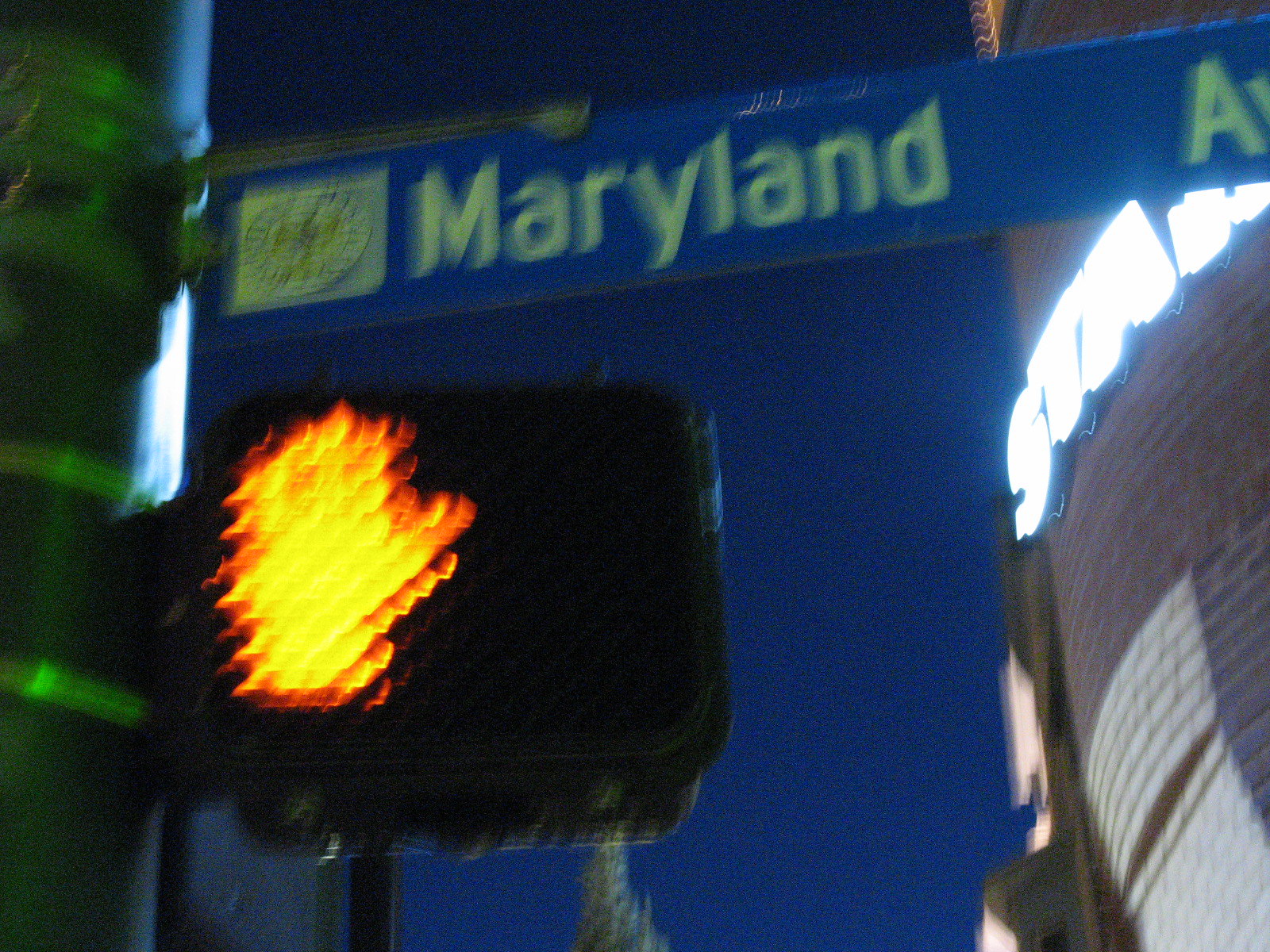Underneath a dark, nighttime sky, an image captures an upward view of an urban crosswalk scene. A prominent crosswalk signal displays a red hand inside a black square box, cautioning pedestrians to halt. Adjacent to the signal, a large blue street sign angles into view, reading "Maryland Avenue" in bold white letters. The sign features a small square logo in its left corner. To the right, a tall building comes into focus, its name partially visible due to bright neon lights displaying the letters "STA." The scene is anchored by a dark metal pole, which not only supports the crosswalk light and street sign but is also secured with metal clasps, visible to the careful observer.